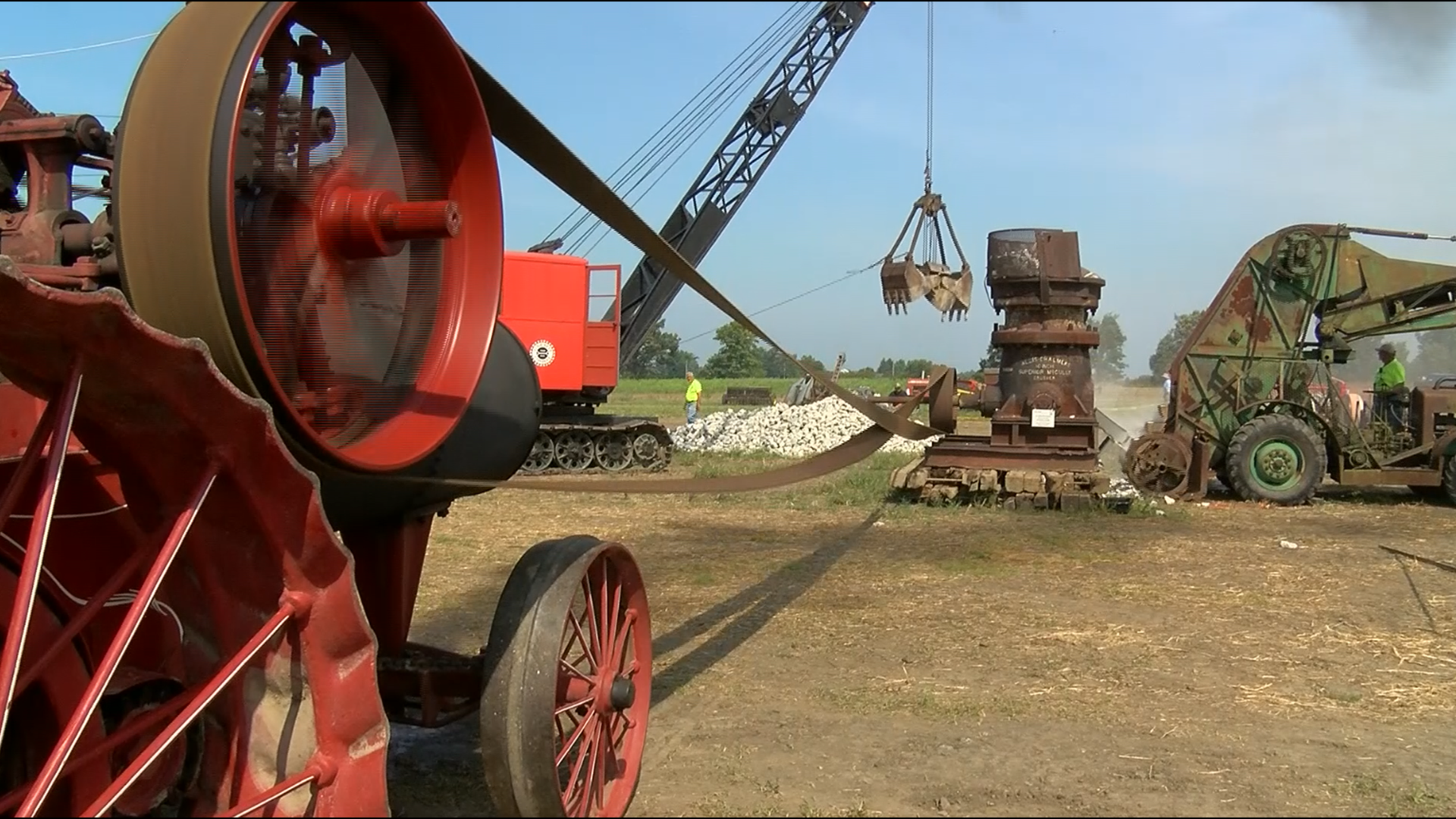This color photograph depicts a landscape-oriented outdoor scene featuring an assembly of early 20th-century industrial machinery, possibly from the 1910s or 1920s, engaged in a collaborative project likely involving rock crushing or heavy construction work. In the distant background stands a vintage crane, its claw attachment dangling halfway down a rope, appearing to lift or lower materials, perhaps white stones, into or out of a pit. Dominating the foreground is another sizable machine equipped with a large pulley system, around which a long belt is wound. This belt extends across the image to a second machine, enabling its operation. On the right-hand side, a third, somewhat ambiguous piece of equipment is present; it is sizable and controlled by a man in a white baseball cap and yellow shirt, which contrasts with the antique nature of the machinery. The overall scene takes place in what resembles a large outdoor theater or a field, bordered by trees, and presents a rare glimpse into historical machinery at work with vibrant, period-defining colors, predominantly red, capturing the rust and age.